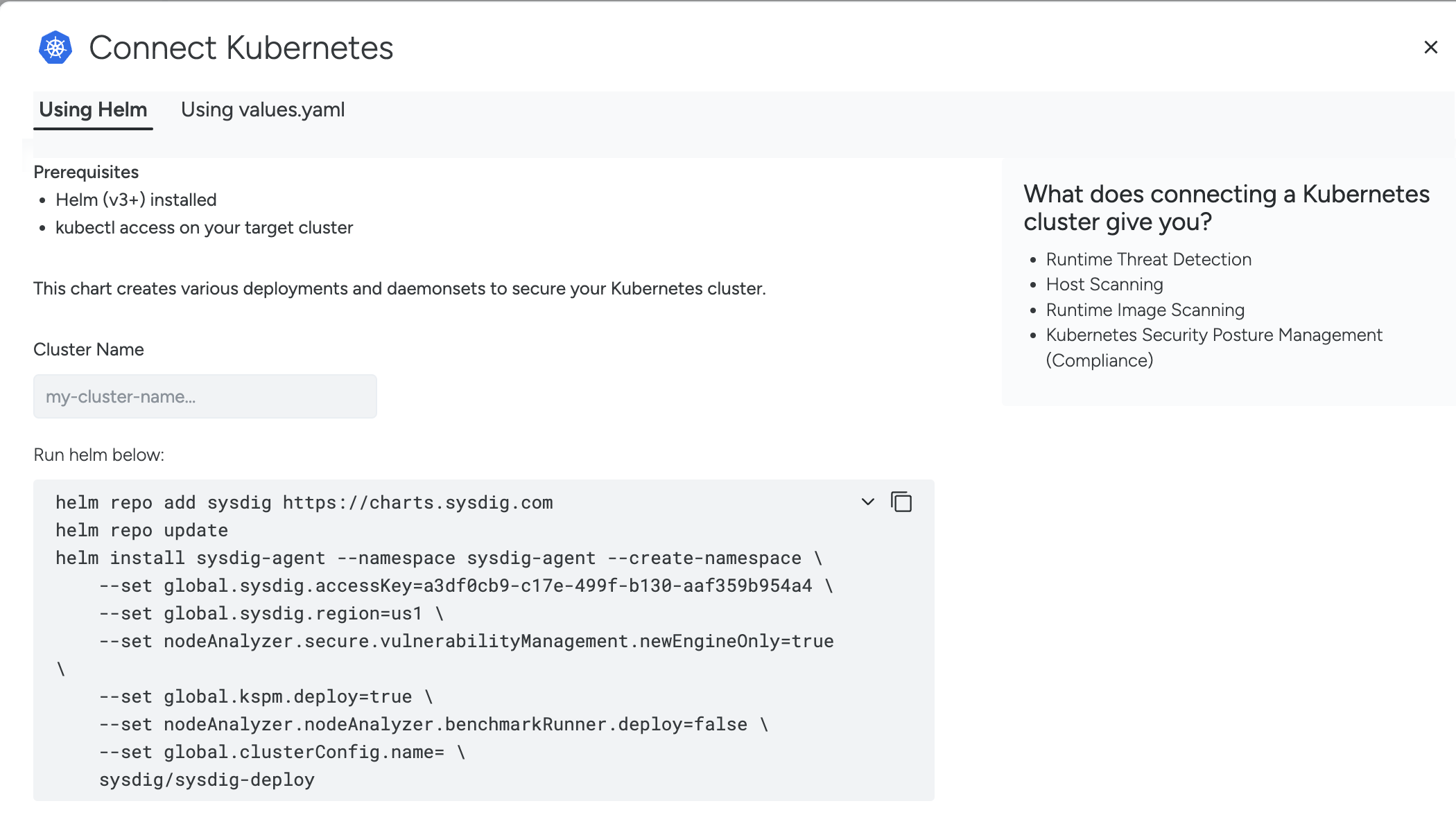Below is a detailed and cleaned-up caption for the image as described:

---

The image appears to be a screenshot of a webpage. At the top, there is a thin white line acting as a border, while the other three sides are borderless, enclosing a slightly gray space. Prominently displayed in blue with a white design is the icon for "Connect Kubernetes." 

To the far right, there is an "X" symbol for closing the window. Below the icon, the text reads "Using Helm," which is underlined, followed by "Using Values.yaml - Prerequisites." It mentions that certain prerequisites need to be installed.

The text then explains that "This chart creates various deployments and daemon sets to secure your Kubernetes cluster." There is a section labeled "Cluster Name" with a space provided for the user to input the cluster name, followed by some code.

On the right side, there's a highlighted section titled "What does connecting a Kubernetes cluster give you?" with the following bullet points:
- Runtime threat detection
- Host scanning
- Runtime image scanning
- Kubernetes security posture management (compliance).